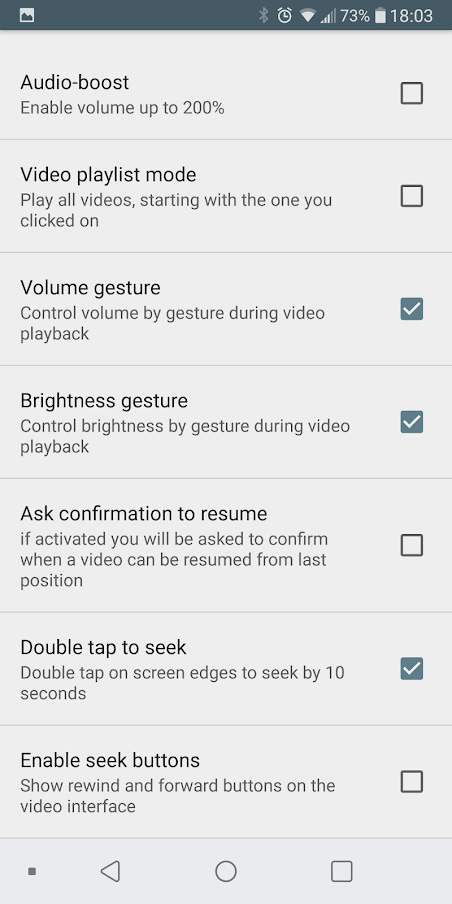Here’s a detailed and cleaned-up caption for the described image:

---

The image depicts a mobile device screen, most likely a cell phone, showcasing a settings menu. At the top of the screen, there is a dark green bar, reminiscent of a teal color, indicating various status icons. On the far left of this bar, a small graphic can be seen. Moving right, there are symbols for Bluetooth, an alarm clock, a strong Wi-Fi connection, followed by a battery icon showing three out of five bars (indicating 73% battery life), and the time displayed as 18:03.

Below this status bar, a settings menu is listed with multiple options, each accompanied by a checkbox to its left. The detailed options are as follows:

1. **Audio Boost** - Enable volume up to 200% (Checkbox not checked).
2. **Video Playlist Mode** - Play all videos starting with the one you clicked on (Checkbox not checked).
3. **Volume Gesture** - Control volume by gesture during video playback (Checkbox checked).
4. **Brightness Gesture** - Control brightness by gesture during video playback (Checkbox checked).
5. **Ask Confirmation to Resume** - If activated, you will be asked to confirm when a video can be resumed from the last position (Checkbox not checked).
6. **Double Tap to Seek** - Double tap on screen edges to seek by 10 seconds (Checkbox checked).
7. **Enable Seek Buttons** - Show rewind and forward buttons on the video interface (Checkbox not checked).

At the bottom of the screen, a slightly different shade of grey bar houses a navigation panel with icons: a small square on the left (potentially indicating activity status), a back arrow symbol (triangle facing left), a home button (circle in the middle), and a square on the far right to view open apps.

---

This cleaned and detailed caption provides a comprehensive description of the image, finely capturing the essence of the content shown on the mobile device’s screen.